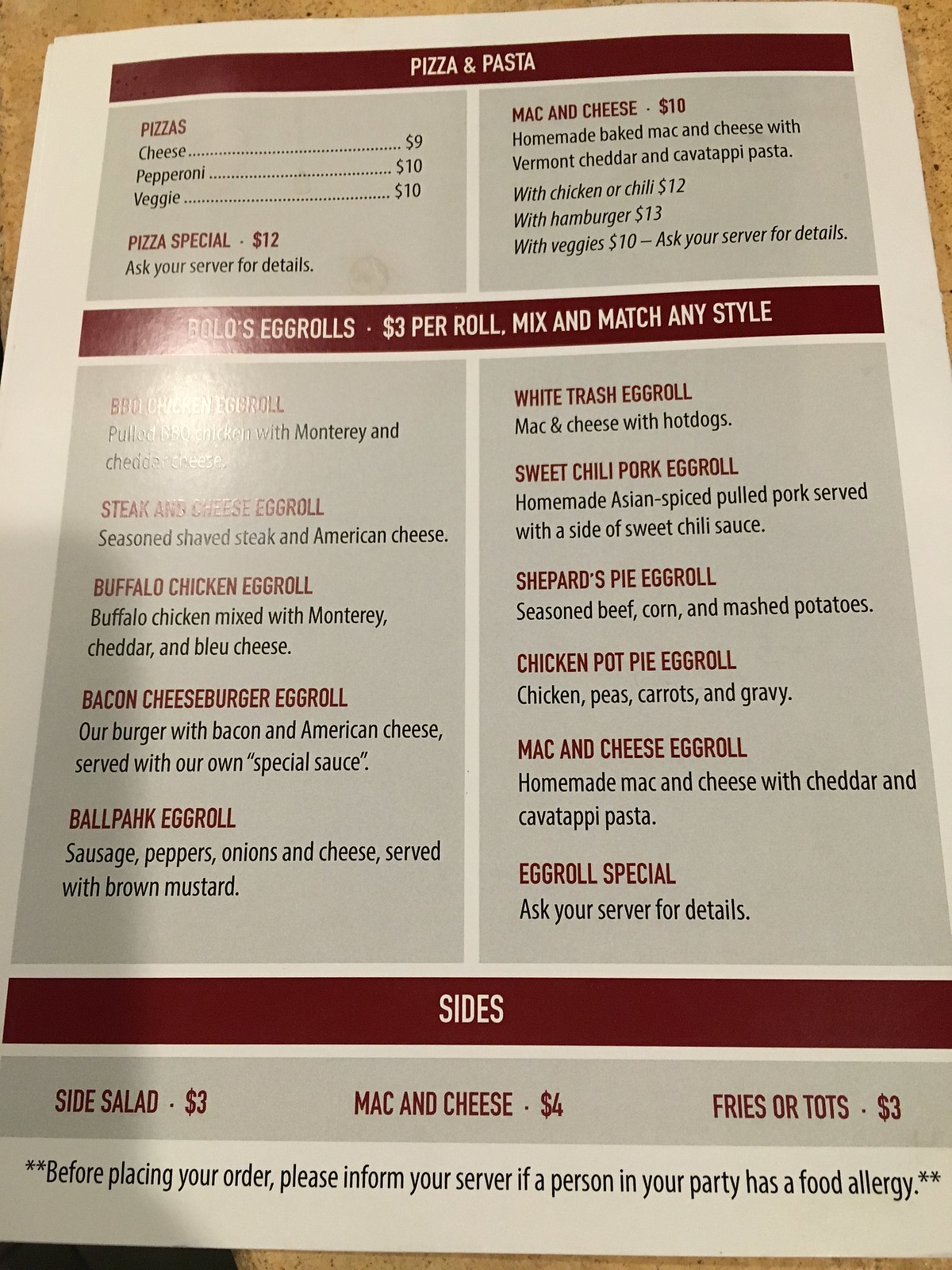This is an image of a photographed restaurant menu. At the top, there's a red line with white text that reads "Pizza and Pasta." Below this heading, listed under "Pizzas," are several options: Cheese Pizza for $9, Pepperoni Pizza for $10, and Veggie Pizza for $10. There’s also a "Pizza Special" for $12, with a note to ask the server for more details.

On the right side, the menu features "Mac and Cheese" priced at $10, described as homemade baked mac and cheese with Vermont cheddar and cavatappi pasta. It offers add-ons like chicken or chili for $12, hamburger for $13, and veggies for $10, again advising to ask the server for details.

Further down, another red line with white text reads "Bolos," followed by "Egg Rolls" priced at $3 per roll, with the option to mix and match any style. Due to a reflection of light, one item is partially obscured; the word "Monterey" is barely legible. 

The legible egg roll options include:
- Steak and Cheese Egg Roll: seasoned shaved steak and American cheese.
- Buffalo Chicken Egg Roll: buffalo chicken mixed with Monterey cheddar and blue cheese.
- Bacon Cheeseburger Egg Roll.
- Ball Park (spelled as "Ball Pock") Egg Roll, humorously noted for a New York accent.
- White Trash Egg Roll.
- Sweet Chili Pork Egg Roll.
- Shepherd's Pie Egg Roll.
- Chicken Pot Pie Egg Roll.
- Mac and Cheese Egg Roll.
- Egg Roll Special.

At the bottom of the menu, another red bar with white text labeled "Sides" lists the following:
- Side Salad for $3.
- Mac and Cheese for $4.
- Fries or Tots for $3.

Lastly, a notice at the bottom reads: "Before placing your order, please inform your server if a person in your party has a food allergy."